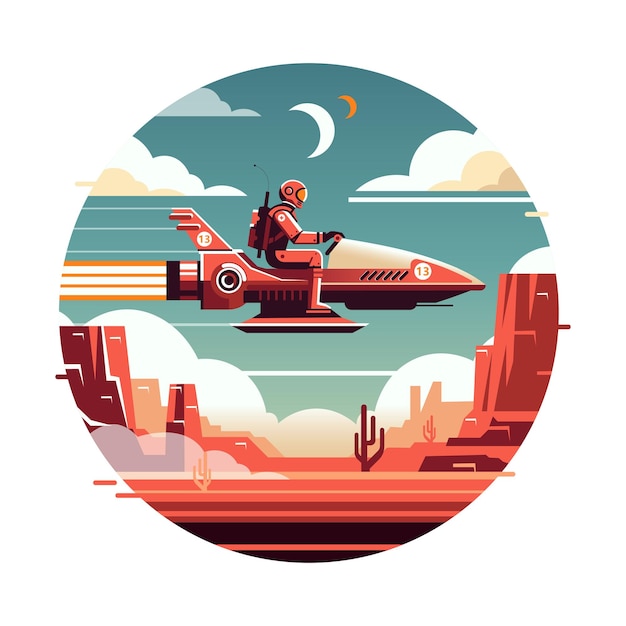This digital print portrays a vibrant, futuristic scene within a circular frame. Dominating the center of the image is a figure in a fully enclosed space suit, complete with a helmet and a fuel pack on their back, riding a horizontally positioned rocket marked with the number 13. The rocket emits a fiery exhaust, suggesting forward motion. The background reveals a striking dichotomy between the upper skies and the lower terrain. 

The sky features various muted blues and greens, dotted with fluffy clouds. On the left, a green cloud floats above a white cloud with a small yellow one in front of it. To the right, a expansive white puffy cloud is accompanied by a pair of yellowish clouds, one being darker khaki yellow. Two crescent moons occupy the sky—one larger and white, the other smaller and gold.

Below this celestial display, a detailed desert scape extends across the bottom of the image in rich reds and oranges. This desert is characterized by cacti and mesa-type structures, emphasizing a rugged, otherworldly ambiance. The vibrant color palette combines tones of red, orange, blue, and green, contributing to the scene's dynamic and vivid nature, and reinforcing the impression of an otherworldly, perhaps extraterrestrial, adventure.